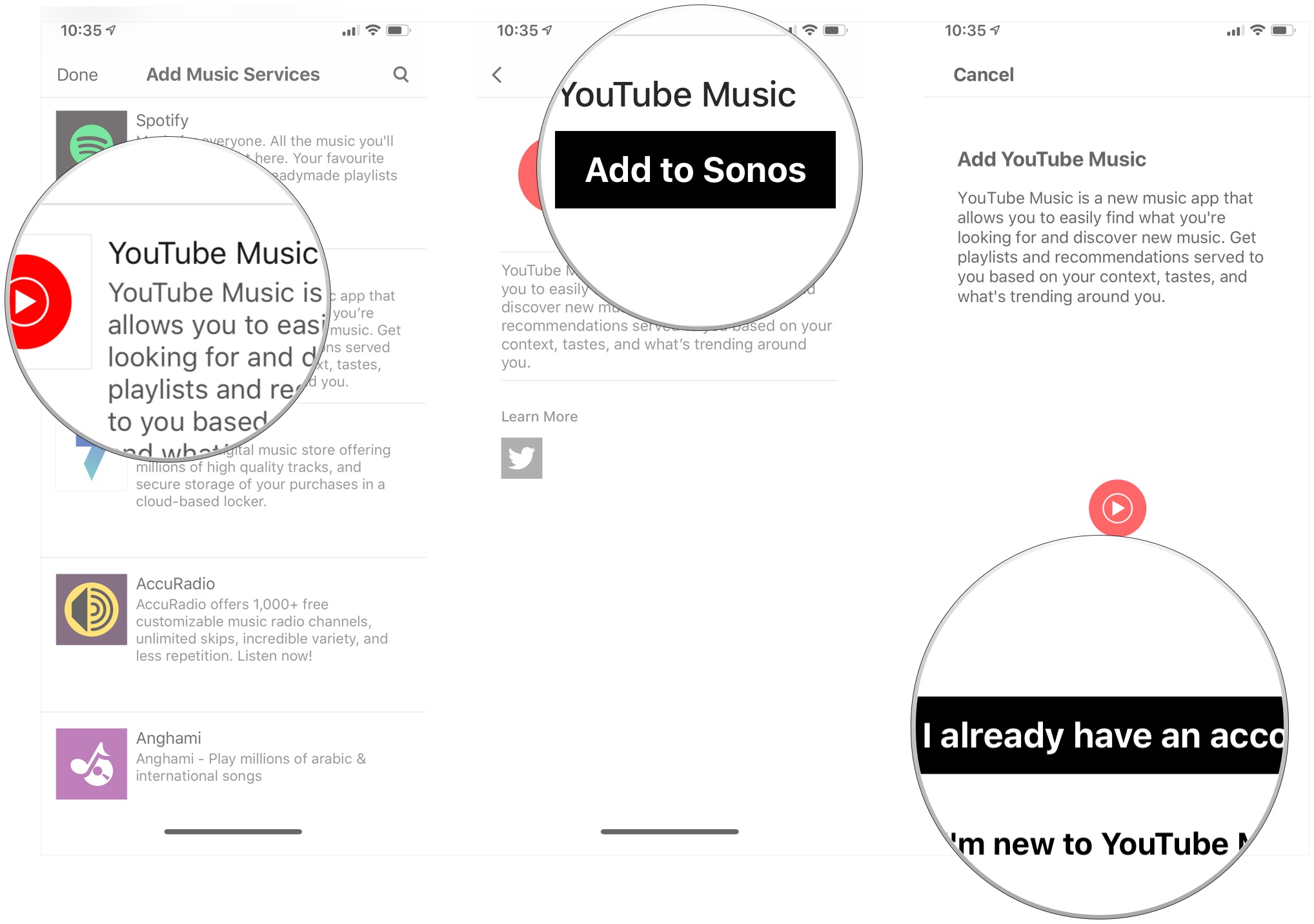This collage consists of three screenshots from a smartphone, meticulously captured side by side.

### General Elements in All Screenshots:
- **Top Row Information**: Each image has a timestamp of "10:35" displayed in the upper left-hand corner. Adjacent to the timestamp is an upward and rightward pointing arrow, followed by a phone signal strength icon showing three out of four bars active, a Wi-Fi signal indicator, and a vertical black battery icon.

### Leftmost Screenshot:
- **Upper Elements**:
  - "Done" is written in the upper left corner.
  - "Add Music Services" is positioned at the top center.
  - A magnifying glass icon symbolizing search is on the top right.

- **Content Below**:
  - A gray box features a green circle with three black lines inside. Next to it is the word "Spotify."
  - This area partially obscures a section below, highlighted by a circle containing larger text with a logo: the YouTube Music logo (a white box with a red circle enclosing a small white circle that has a red play arrow pointing to the right).
  - Text partially visible includes: "YouTube music is..." and "easy... looking for Ann."
  - Lower down, a purple box with a yellow circle shows a horn with sound lines, labeled "AccuRadio."
    - AccuRadio Description: "AccuRadio offers 1,000+ free customizable music radio channels, unlimited skips, incredible variety, and less repetition. Listen Now!"
  - Further below, a lavender box with a white music note and CD icon labeled "Anghami."
    - Anghami Description: "Anghami — play millions of Arabic and international songs."

### Middle Screenshot:
- **Upper Elements**:
  - Text in black reads "YouTube Music."
  
- **Content Below**:
  - Below "YouTube Music" is a black box with white text that reads "Add to Sonos."
  - Description under this box is partially obscured by the overlaid circle.
  - Beneath the description, a "Learn More" link appears.
  - Lower part contains a yellow box with a white Twitter bird logo.

### Rightmost Screenshot:
- **Upper Elements**:
  - "Cancel" is prominently displayed in the upper left corner.
  - Below, "Add YouTube Music" text is seen.

- **Content Below**:
  - "YouTube Music is a new music app that allows you to easily find what you're looking for and discover new music. Get playlists and recommendations served to you based on your context, tastes, and what's trending around you."
  - A gray circle encloses a black bar with partially visible white text: "I already have an account."
  - At the bottom, a text reads "Add New to YouTube."

This compilation of screenshots effectively showcases a mix of various music service options and their associated app functionalities, descriptions, and icons.